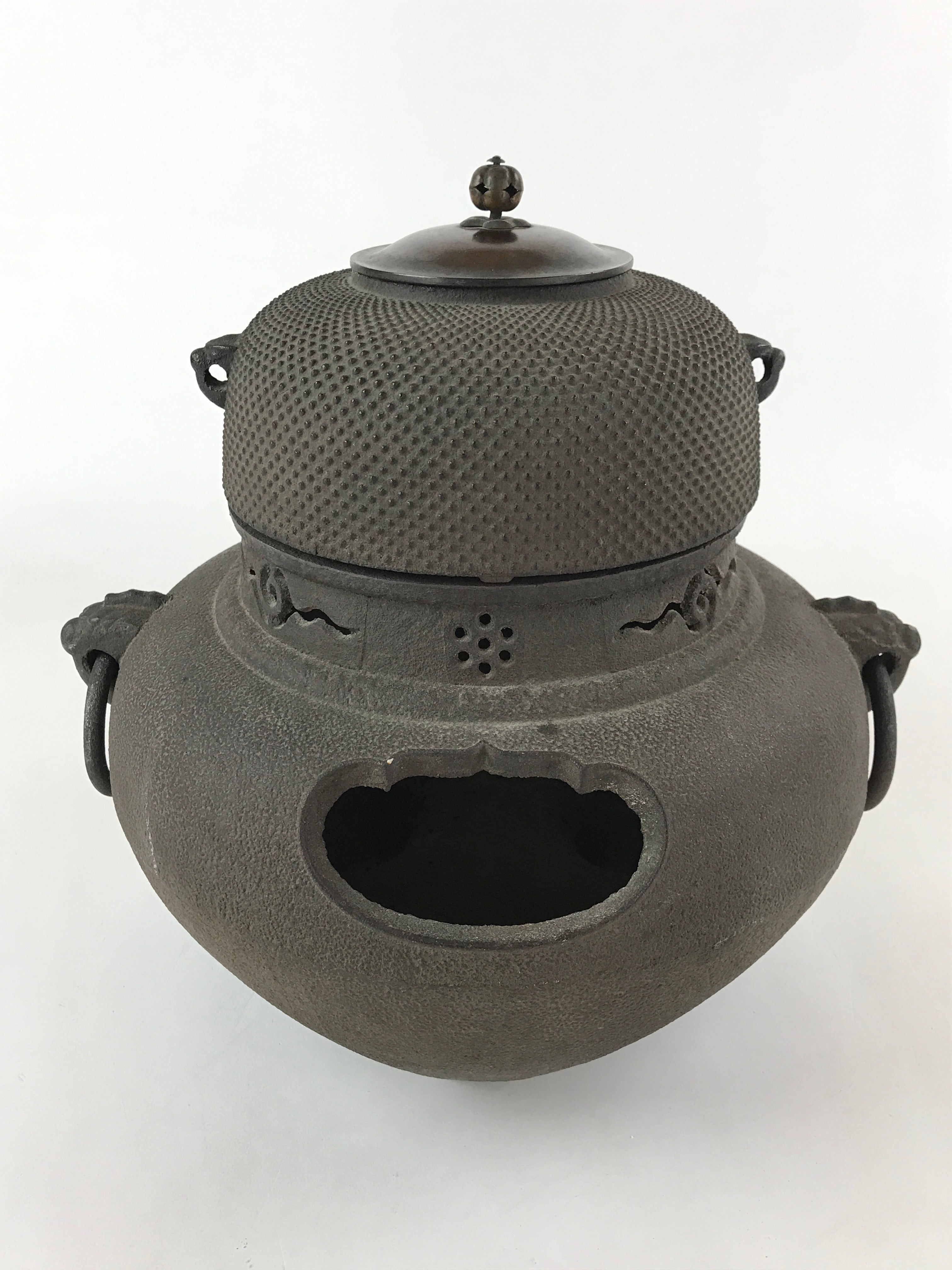The image depicts a small, intricately designed gray kiln or oven set against a light gray to white background. This dome-shaped object features a pot-like base with a large oval opening in the middle, which appears ashy, indicating past use with fire. It has a beady texture with star-patterned dots along the center lining, adding to its detailed craftsmanship. On both sides of the base are two handles, and another pair of small handles are located on the round, stubby lid at the top. The lid, possibly used to release smoke or flames, has a small bulbous metal piece protruding from its center. The structure is vase-like, with multiple openings and slots, suggesting it could function as a multi-purpose pot or kiln for baking or burning.